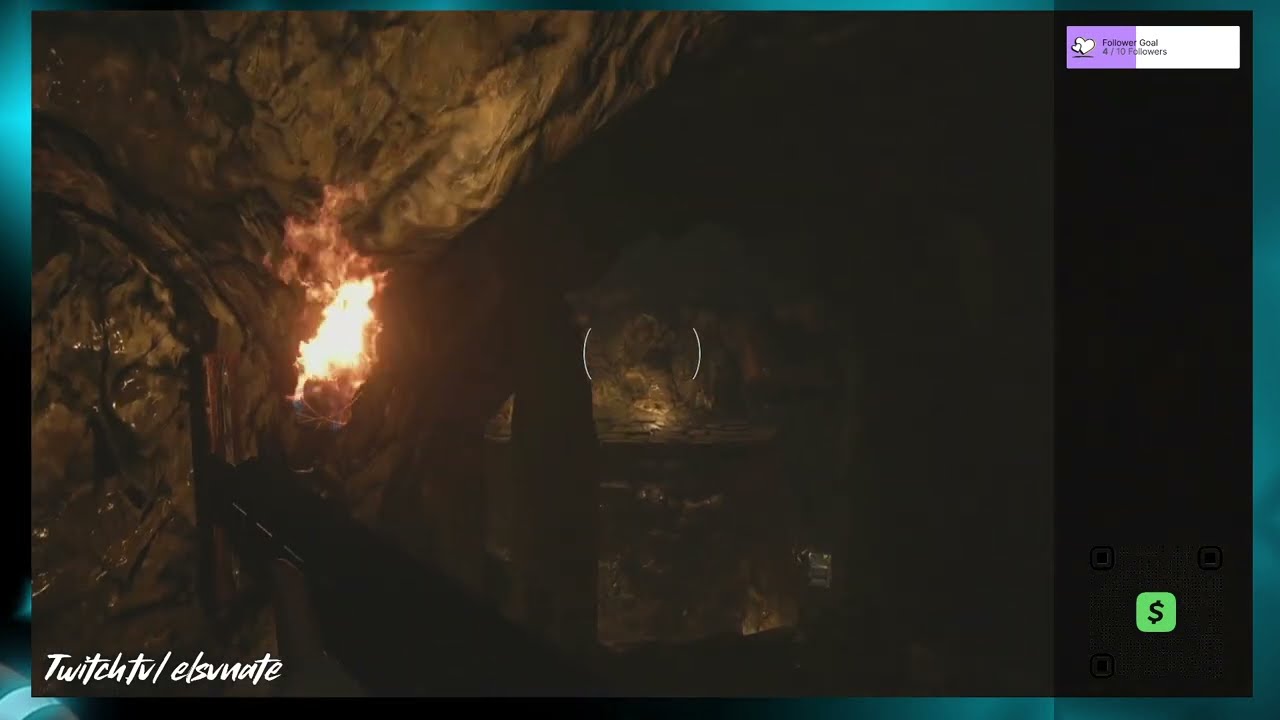This image appears to be a screenshot from a video game, showcasing a dark, shadowy cave scene taken at night. The cave's rocky walls are barely visible, illuminated only by a fire inside the cave that casts a dim glow. In the center of the screen, two white parentheses or reticle-like markers suggest an aiming mechanism typical in video games. Overlaying the image, there is a brightish blue border framing the in-game view. 

In the upper right-hand corner, a partially filled purple box indicates a follower goal of "4 out of 10 followers." The bottom right-hand corner features a green square with a dollar sign, presumably the Cash App symbol. Along the bottom left corner of the screen, text reads "twitch.tv/elsvnate," identifying the streaming platform and the user's channel. Additionally, the left corner has some unclear white text that could be "Twitch toll estimate." Overall, the image is quite dark with little visible detail outside the illuminated areas.